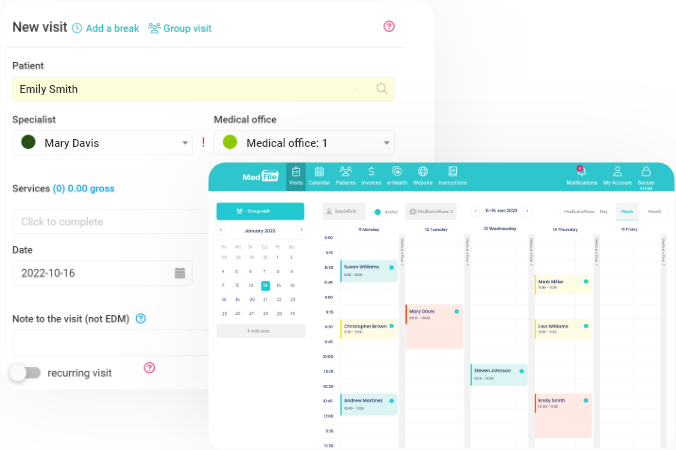In the foreground of the image, there is a primary interface window partially overlapped by a smaller pop-up box. The primary window seems to be an organizational tool, potentially a calendar or schedule manager. The header of this window features a turquoise bar that contains several tabs labeled "Visits," "Calendar," and others that are too small to read clearly. Below the header, on the right side, there are icons including a bell with a notification indicator suggesting one new notification, a digital avatar representing user profile access labeled "My Account," and a lock icon marked "Secure."

On the left-hand side within this primary interface, a calendar view displays the month of January 2022. The specific date of January 14th is highlighted with a blue box. Adjacent to this calendar display, the detailed weekly schedule spans the entire week, breaking down appointments or events by time slots starting at 8 AM. Each scheduled item is visually distinguished by colored boxes (e.g., blue, red, or orange) and is annotated with the event title and time in bold black text.

The pop-up box, partially covering the main interface, is possibly an input form or additional details for the event being managed on the calendar. It adds another layer of interactivity to the scene, suggesting an active engagement with the scheduling tool.